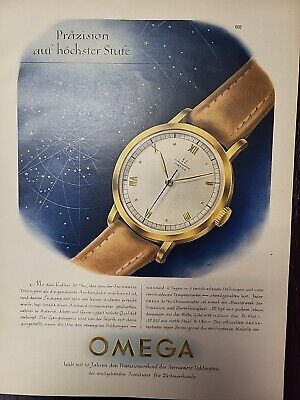The image is a vintage magazine advertisement for an Omega watch. It features an elegant illustration of the timepiece, highlighting a luxurious design with a gold frame and a white face adorned with gold Roman numerals marking the hours at 12, 2, 5, 6, 7, and 10. The watch is complemented by a sophisticated brown leather band. The background of the advertisement is a captivating blue, embellished with stars and astrological constellations, lending a celestial aura to the scene. The top left corner of the image bears the words “Precision and Horster Strut” or “Precision and Honcher Suit,” though the exact phrase might vary slightly and is in a foreign language. Below the watch, at the bottom of the ad, is the brand name "Omega" in a distinguished gold font. The advertisement also includes two columns of descriptive text, presumably in a foreign language, detailing the features of the watch, although the small font size renders the text unreadable. The entire image provides a sense of luxury and timeless precision, typical of Omega’s branding.